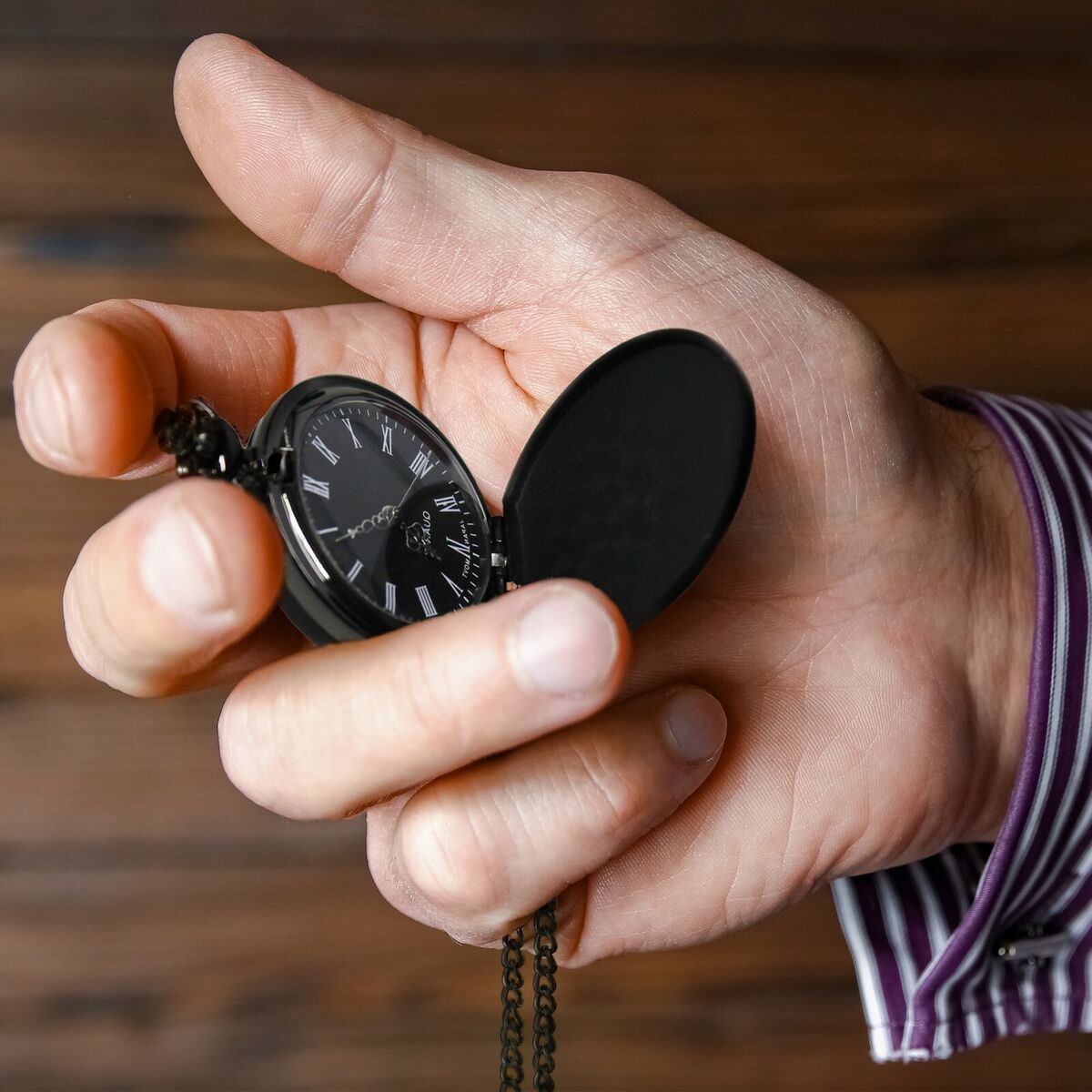In this detailed, realistic photograph, a close-up view of a man's right hand dominates the center of the square frame. The skin tone is white, and the hand appears somewhat thick, hinting at a male subject. His thumb is pointing upwards, revealing the palm. The wrist is adorned with the cuff of a purple and white striped dress shirt, complete with a visible cuff link.

The man is clutching an open black pocket watch with a black case and frame in his hand. The face of the watch is also black, featuring white Roman numerals to indicate the different times, and stainless steel pointer arms. Extending from the pocket watch is a black chain link that drapes downward. The exact time displayed on the watch face appears to be around 10 minutes to 10.

Behind the hand, the background is softly blurred but suggests the presence of brown wooden plank walls. This out-of-focus setting enhances the sharpness and clarity of the hand and watch, drawing attention to their intricate details and the poised positioning of the hand as if preparing to press the timer.